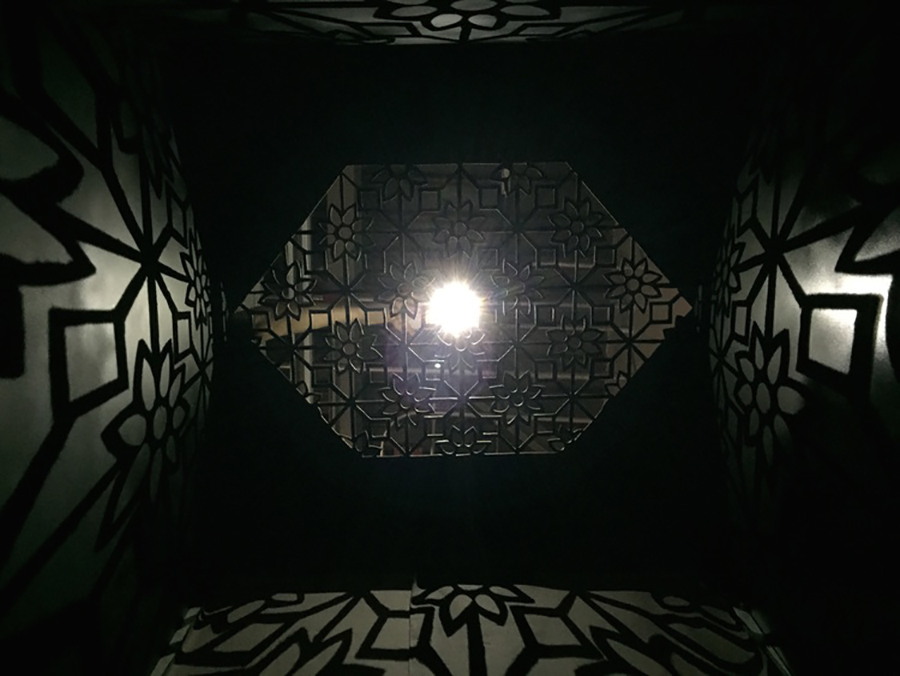This photograph captures the interior of a dark room with black walls and a gray cement floor. At the center of the image, there is an intricate, hexagonal lattice design that combines geometric and floral motifs, bordered by black bars and forming a square with triangular sides. A bright light shines through this latticework, projecting highly detailed shadows of the design onto the surrounding walls and floor. The interplay of light and shadow creates a striking pattern, with flowers and geometric shapes clearly visible in the projections. The overall effect is as if the viewer is looking up through an ornate aperture in a confessional or a similarly enclosed space, highlighting the dazzling complexity of the design illuminated against the otherwise dark environment.